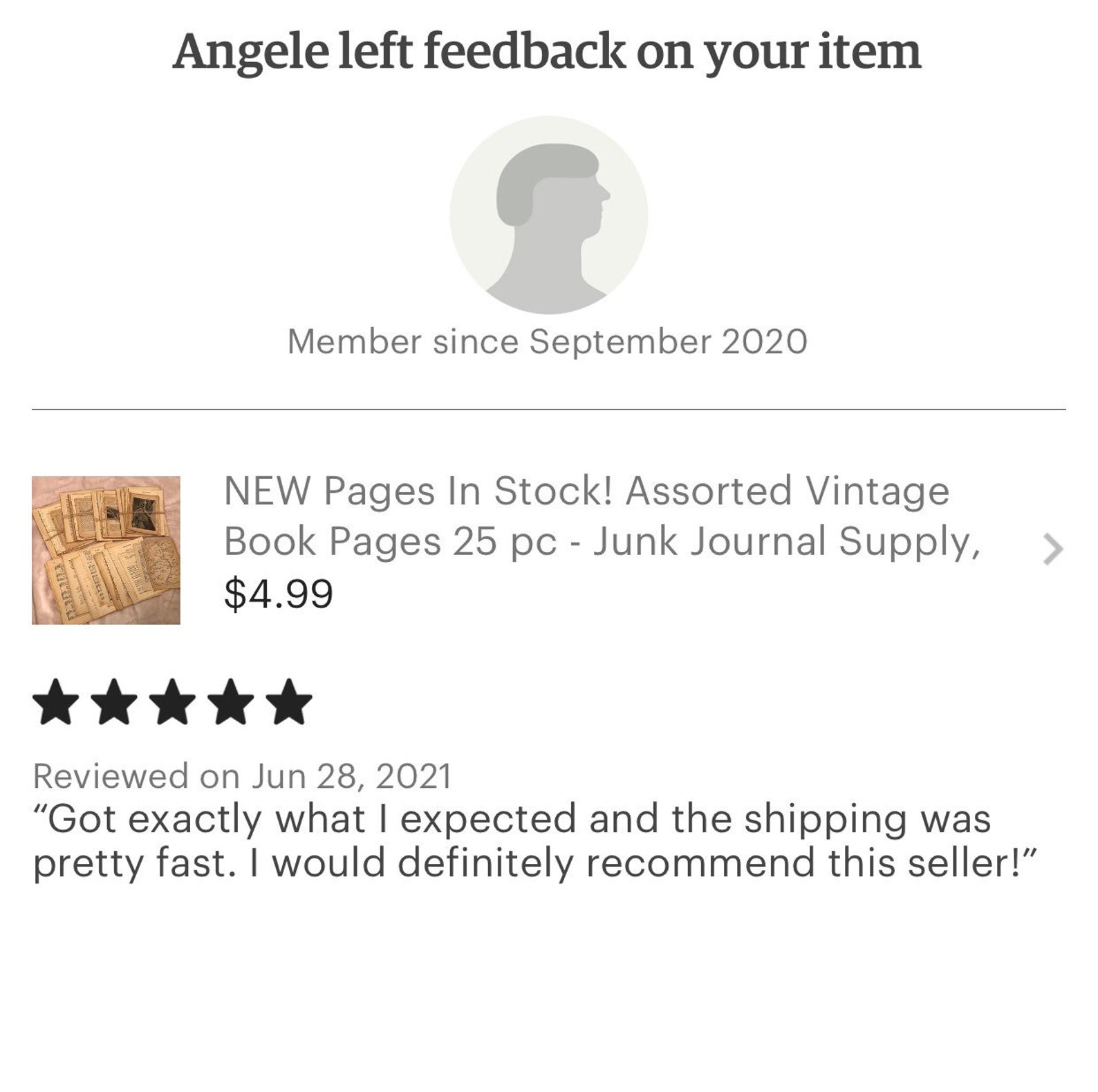Screenshot of a customer review with a white background, divided into two sections. 

The top section features the following:
- Centered at the very top, in bold letters: "ANGELE"
- Underneath, the text: "Angeli left feedback on your item"
- Below that is a person’s avatar with the text in gray: "Member since September 2020"

A gray line separates the top section from the bottom section.

The bottom section includes:
- On the left, an image of the items listed for sale: "New pages in stock, assorted vintage book pages, 25 pieces, junk journal supply"
- The price: "$4.99"
- A five-star rating
- The review date: "Reviewed on June 28th 2021"
- The customer's feedback: "Got exactly what I expected and the shipping was pretty fast. I would definitely recommend this seller."

The overall context suggests this is feedback from a satisfied customer on a sales platform, likely eBay, reviewing a transaction and expressing satisfaction with the product and delivery speed.